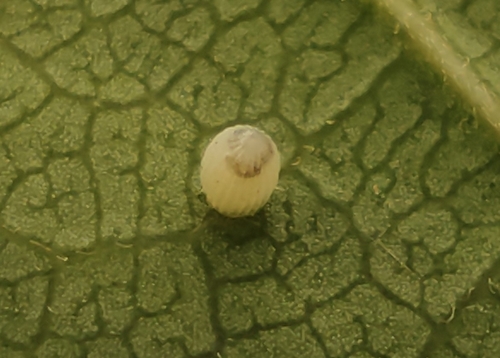This is a highly magnified, extreme close-up view of a green leaf's surface, resembling the leathery pattern of wrinkles similar to those seen on a brain. You can see the intricate, irregular sections that comprise the leaf's texture, with light green areas and darker green veins crisscrossing it. On the right side of the image, the stem is visible, leading our eyes to the central feature of the photograph: a small, white spore or insect egg, standing about a quarter inch tall and wide. This growth has white ridges running vertically along its body and is capped with a brownish-tan spot at its peak. The detailed, top-down view reveals the complexity of the leaf's structure and the mysterious nature of the tiny spore-like object affixed to it.